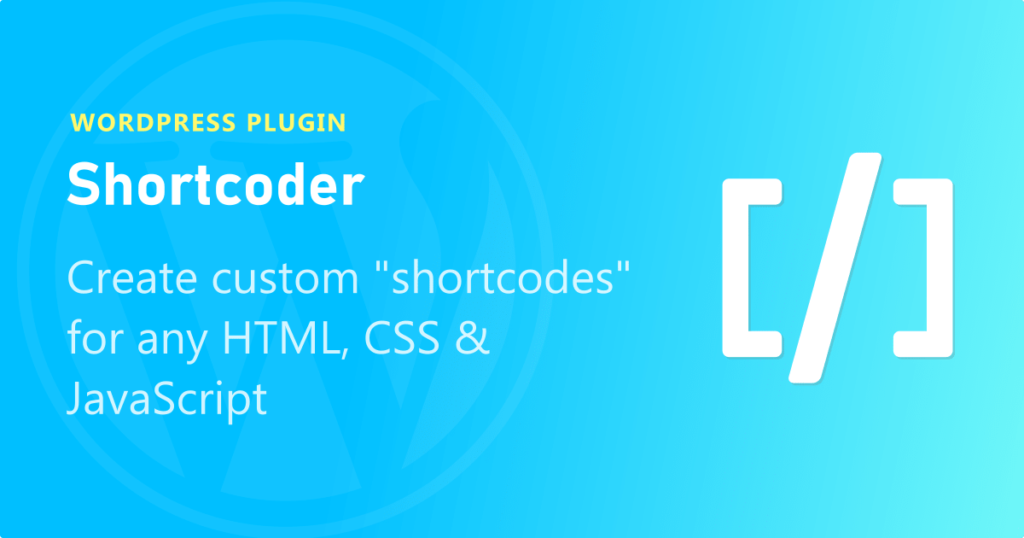The image depicts a vibrant and aesthetically pleasing website featuring a bright and inviting color scheme of light blue hues that resemble teal, evoking the tranquil appearance of an ocean. In the background, there is a subtle, almost ethereal large circle on the left side, which encloses a faintly discernible image. 

At the upper left-hand corner, the text "WordPress Plugin" is prominently displayed in yellow. Directly beneath this, "Shortcoder" is written in large, bold white letters. Further below, the description "Create custom shortcodes (for any HTML, CSS, and JavaScript)" is provided, clearly communicating the functionality of the plugin.

On the right side of the image, where the blue tones transition to a lighter shade reminiscent of tropical waters, there is a stylized letter "C." This "C" has a boxy appearance, akin to a bracket, with a diagonal line running from its top-right to bottom-left. Adjacent to it, a mirror image of the "C" is present, which also resembles a bracket. Both these elements, the line and the brackets, are depicted with a pronounced thickness, adding a sense of boldness and structure to the design.